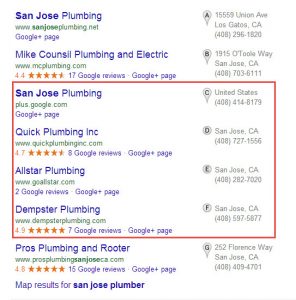The image displays a set of Google search results on a white background. The top result is for "San Jose Plumbing," with the corresponding website URL listed as "www.sanjoseplumbing.net." Directly beneath this, there is a blue hyperlink directing users to the business's Google Plus page. To the right of this information, a pushpin icon marked with an 'A' indicates the business's location at 15550 Union Avenue, Los Gatos, California, 48296-1820.

The second search result is for "Mike Council Plumbing and Electric," featuring the URL "www.mcplumbing.com." This business has a rating of 4.4 stars out of 5 based on 17 Google reviews, with a blue hyperlink to its Google Plus page as well. The address provided for Mike Council Plumbing and Electric is 1915 O'Toole Way, San Jose, California, 48703-611.

Below these entries, there is a large red square highlighting an area that contains information on four different businesses, including their names, addresses, and phone numbers.